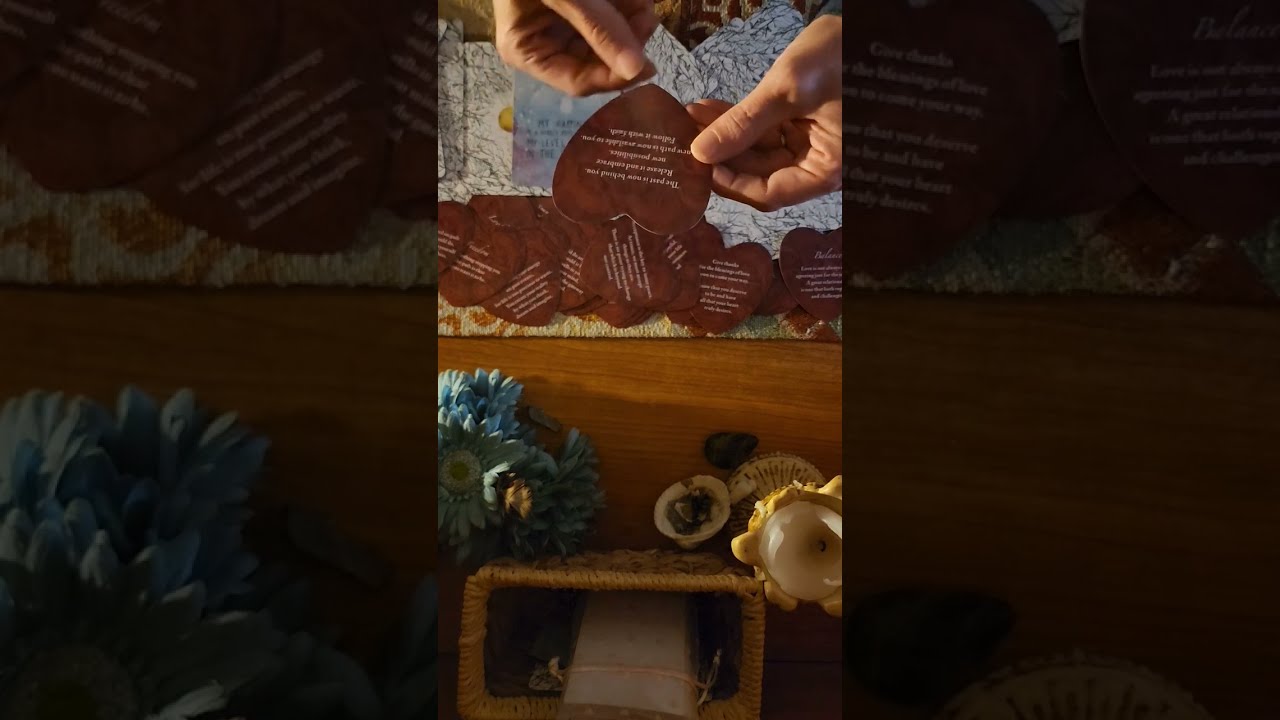The image is a top-down view of a wooden tabletop, split into two distinct halves. In the upper half, two slightly older hands hold a brown, upside-down paper heart adorned with white text, surrounded by many similar paper hearts, suggesting they are being crafted to pass out. The person's thumb is on top of the heart, with fingers gently cupping it from beneath, while another hand, slightly blurred, is positioned to the side. Below the hands, there are additional decorated cards featuring black-and-white leaf patterns.

The bottom half of the image reveals a more open area of the table, which hosts an assortment of items: a blue flower to the left, a partially melted white candle in a holder, and a rounded shell-like container holding what appears to be paper or wick material. On the lower-left corner, a wicker basket contains more paper. The right side of this half is marked by a zoomed-in section with a light gray tint, adding a unique layer to the composition.